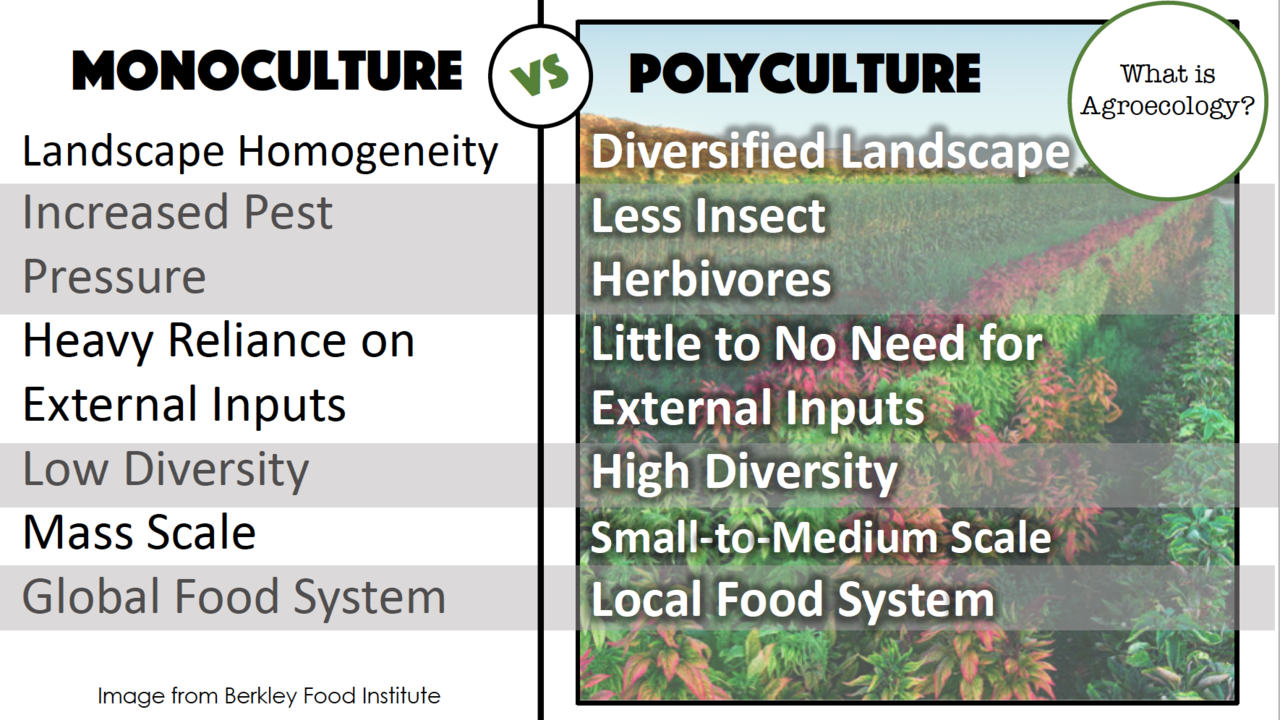The image is an informational slide comparing monoculture and polyculture in the context of agroecology. The slide is divided into two sections. On the left side, with a white and gray alternating background, it says "Monoculture" in large black font at the top. Below "Monoculture," a column lists the characteristics: landscape homogeneity, increased pest pressure, heavy reliance on external inputs, low diversity, mass scale, and global food system. 

In the middle of the slide, the word "versus" indicates the contrast. On the right side, overlaid on a colorful photograph of a diverse field of flowers, it says "Polyculture" in a similar column format. The column lists: diversified landscape, less insect herbivores, little to no need for external inputs, high diversity, small to medium scale, and local food system. 

A white circle in the upper right corner of the image poses the question, "What is agroecology?", while the bottom left note attributes the image to the Berkeley Food Institute. The overall impression strongly favors the benefits of polyculture over monoculture.